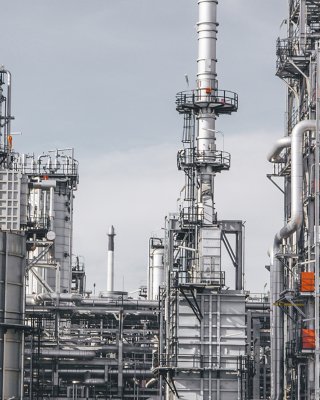This black and white photograph captures a sprawling industrial plant characterized by a complex web of metal structures. Prominent in the scene are steel towers and a labyrinth of pipes weaving their way horizontally, vertically, and in zigzag patterns. Dominating the right side is a cylindrical tower that stretches from the ground to the top of the image, gradually tapering and adorned with circular, black metal balconies or crow's nests, reminiscent of those on a pirate ship. These balconies are equipped with railings, suggesting access for maintenance purposes. The left side features another tall, white cylindrical tower, also enmeshed with an array of pipes, including three protruding from its top. The foreground is filled with a dense wall of pipes and steel beams, creating a textured, industrial tapestry that ascends to the middle of the photo. The entire scene is enveloped in shades of grey, from the metallic components to the overcast sky with white clouds, reinforcing the stark, utilitarian atmosphere of this enigmatic factory-like plant seen often along routes like the New Jersey Turnpike.